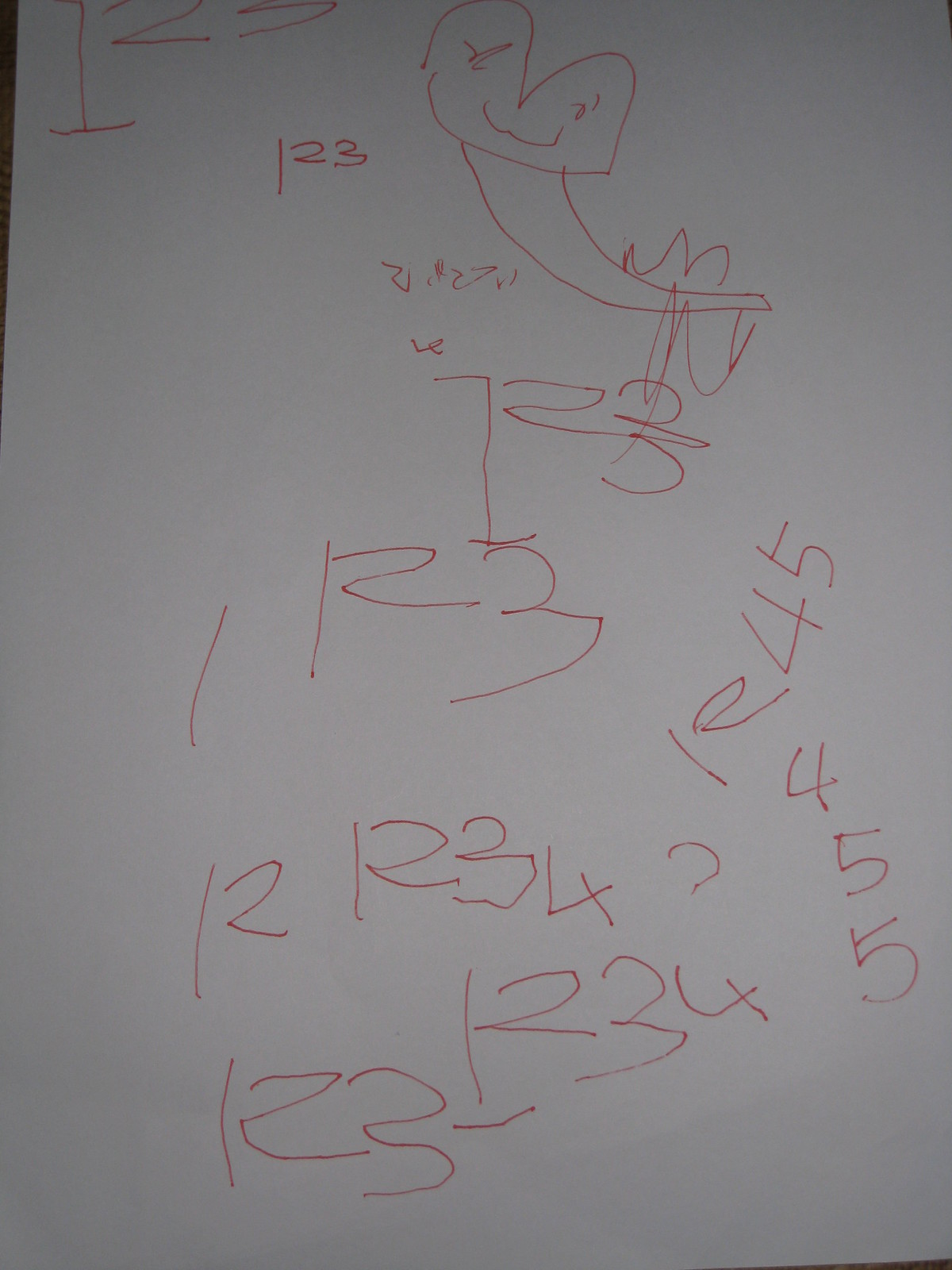This image showcases a sheet of plain white paper adorned with childlike drawings and numbers, created using a simple red pen. Starting from the bottom of the page, there are sequences of numbers, specifically "1, 2, 3" followed by another sequence "1, 2, 3, 4, 5," written in a playful, inexperienced handwriting indicative of a beginner's efforts. The numbers are arranged in a roughly vertical line, contributing to the overall haphazard yet endearing aesthetic.

At the top of the page, the focal point is a whimsical drawing that resembles an "M" shaped figure. This creative design features eyes positioned on each curve of the "M," with a cheerful smile beneath, giving the impression of a friendly face. The ends of the "M" are connected by a line, which also includes a smiley face, further enhancing the playful theme. Two lines extend from this face, curving from the left side toward the center, suggesting the outline of a tail and adding a sense of animated motion to the doodle. The illustration and handwritten numbers together create a charming snapshot of early childhood artistry and experimentation.